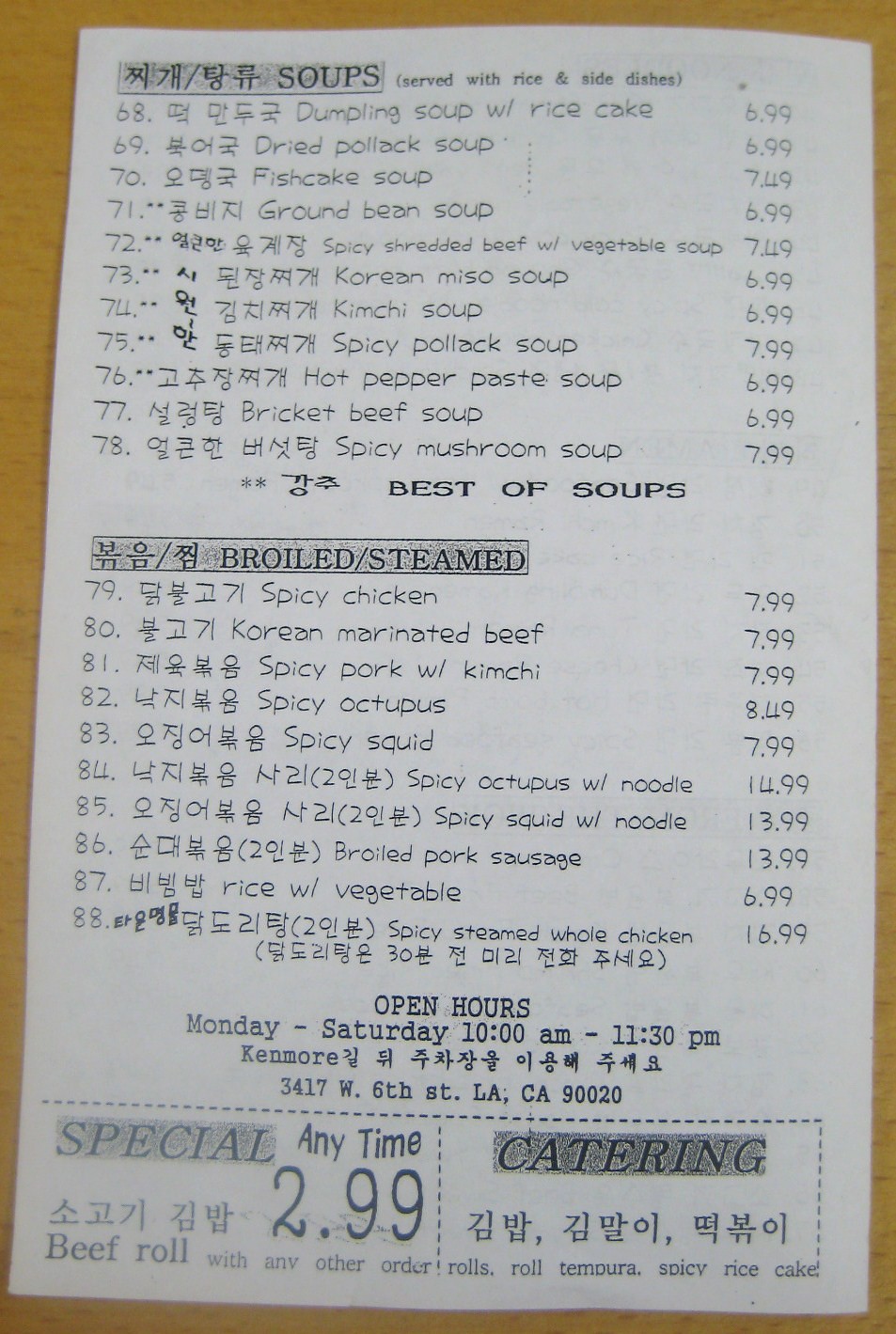The image is a detailed close-up of a restaurant menu, displaying various Korean dishes with their corresponding prices. The menu is printed in black text on a white piece of paper and is positioned on a wooden surface. The dishes are listed sequentially with their respective numbers and prices, as follows:

- 68. Dumpling Soup with Rice Cakes $6.99
  *Note: Soups are served with rice and side dishes.*
- 69. Dried Pollack Soup $6.99
- 70. Fish Cake Soup $7.49
- 71. Ground Bean Soup $6.99
- 72. Spicy Shredded Beef with Vegetable Soup $7.49
- 73. Korean Miso Soup $6.99
- 74. Kimchi Soup $6.99
- 75. Spicy Pollack Soup $7.99
- 76. Hot Pepper Paste Soup $6.99
- 77. Briquette Beef Soup $6.99
- 78. Spicy Mushroom Soup $7.99

Underneath these listings, there is a category titled "Best of Soups" followed by "Broiled/Steamed," and more dishes are listed:

- 79. Spicy Chicken $7.99
- 80. Korean Marinated Beef $7.99
- 81. Spicy Pork with Kimchi $7.99
- 82. Spicy Octopus $8.49
- 83. Spicy Squid $7.99
- 84. Spicy Octopus with Noodle $14.99
- 85. Spicy Squid with Noodle $13.99
- 86. Broiled Pork Sausage $13.99
- 87. Rice with Vegetable $6.99
- 88. Spicy Steamed Whole Chicken $16.99

The menu also provides the restaurant's operating hours and location details at the bottom:

- Open Hours: Monday through Saturday, 10 a.m. to 11:30 p.m.
- Address: 3417 West 6th Street, Los Angeles, California 90020

In the bottom left corner of the menu, there is a special offer highlighted:
- "Special Anytime: $2.99 Beef Roll with any other order."
- "Catering Rolls: Roll Tempura and Spicy Rice Cake."